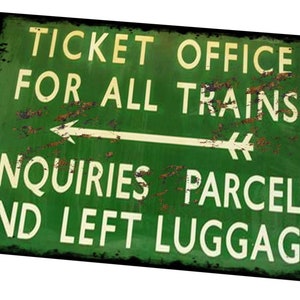The image depicts a heavily weathered and aged rectangular metal sign, measuring about two inches in width and one and a half inches in height, with a slightly tilted angle—its upper left-hand corner higher than the rest. The background of the sign is a faded green, marred with rust and dirt, particularly prominent over the word "TRAINS," and complemented with a black border starting to corrode. The sign's white capital lettering has yellowed with time, reading "TICKET OFFICE FOR ALL TRAINS" in two prominent rows at the top. At the center, an arrow, marked by slanted lines on its right side, points to the left. Below the arrow, partially obscured, the text reads "ENQUIRIES, PARCEL, AND LEFT LUGGAGE," with missing letters: the “I” in "ENQUIRIES," the “A” in "AND," and the “E” in "LUGGAGE." The sign's surface is further marred by various scrapes, suggesting past bumps or impacts.